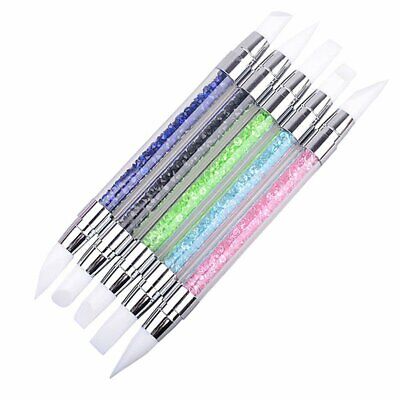This photograph features five sleek, futuristic-looking instruments with a design that suggests they might be upscale pens or applicating tools. Each item is distinguished by a chrome-like cap at both ends, enclosing a white rubber tip that remains unused. The handles of these instruments are filled with different colored bead-like materials, giving them a glittery appearance. From left to right, the colors inside the handles are dark blue, black, bright green, light blue (cyan), and bright pink (or bubblegum pink). The instruments are aligned diagonally across a white background, positioned at an angle that suggests a 40-degree tilt or from a 2 o'clock to 8 o'clock orientation. The exact function of these instruments is not specified, suggesting they could be for writing, painting, or perhaps nail art.